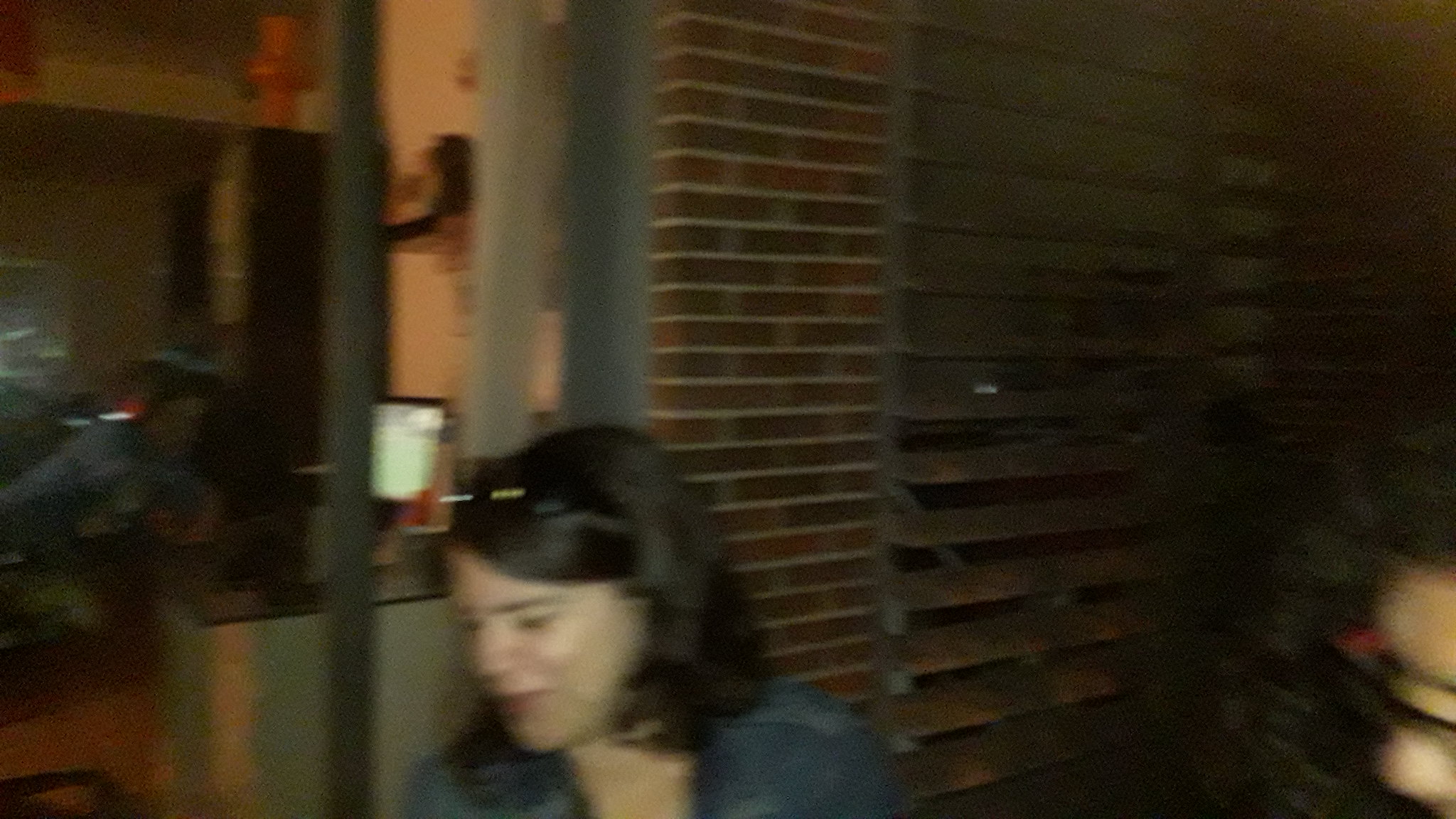In this image, a young Caucasian woman, likely in her late 20s with brunette hair styled in a short bob and side bangs, is prominently featured outside a home. She is wearing a blue jean shirt or jacket and has sunglasses perched atop her head. Her smiling expression suggests a relaxed and pleasant demeanor. Next to her, another figure, presumably a man, is also present but is mostly obscured. The background reveals various elements of the home’s exterior and interior. To the right of the woman, there is a window with wooden blinds, some of which are partially open, offering a glimpse inside the home. Inside, a living room with a couch and curtains is visible, along with what appears to be a desk holding a computer monitor and possibly a hat hanging nearby. In the backdrop, a red brick pillar or column stands alongside some gray concrete, hinting at the structural elements of the house. The setting seems to capture the casual atmosphere of an evening, possibly outside a shop or small restaurant, given the details of the shutters and the scene's overall ambiance.